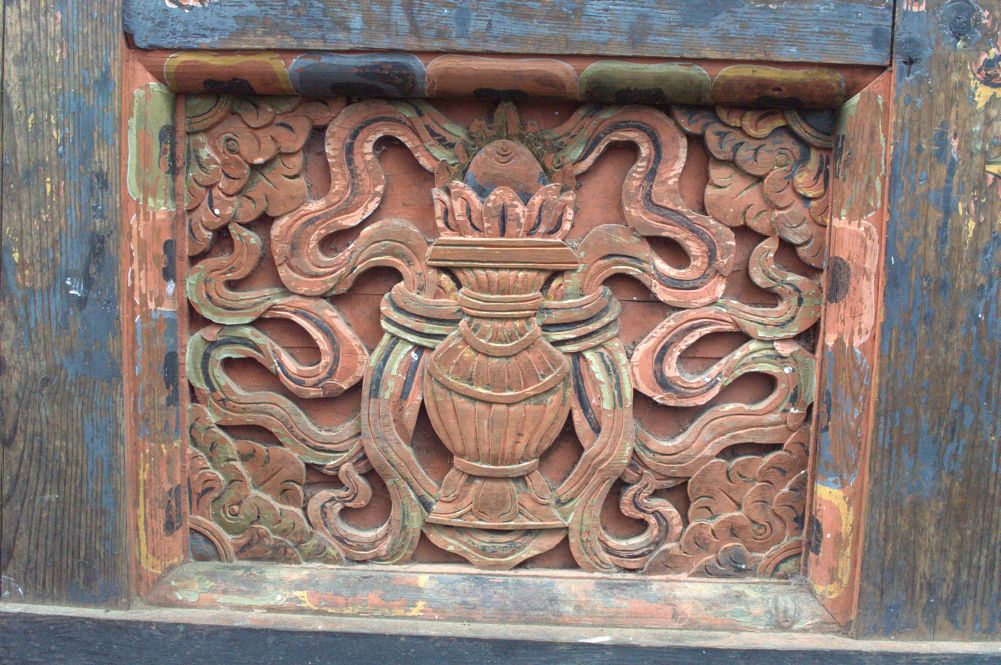The image depicts a rustic, intricately carved wooden art piece, seemingly part of a larger wooden structure such as a gate, doorway, or piece of furniture. At the center of the design is an ornate terracotta-colored vase, from which numerous swirling, snake-like lines extend outward, reminiscent of a sea monster's hair. These lines and the vase itself form the focal point of the carving, surrounded by ornate designs that include cloud-like motifs at each corner. The wooden frame encasing the artwork features a multicolored inset with hues of blue, green, yellow, and terracotta, while the frame itself is predominantly worn and has large splotches of light blue paint, suggesting significant age. The overall color palette and detailed craftsmanship emphasize the piece’s historical and artistic value.